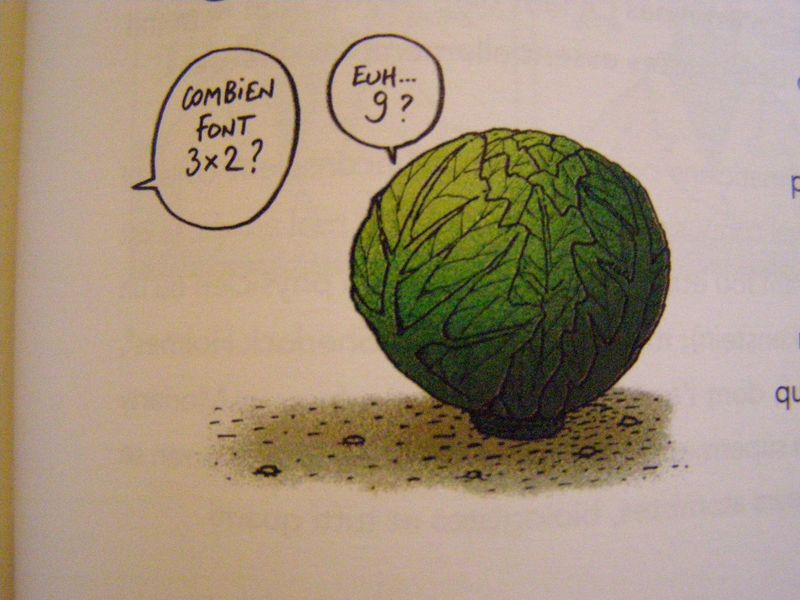This image features a detailed drawing of a brussels sprout, positioned on a white piece of paper which bears faint traces of black text on the other side. The sprout is depicted with a green, round, almost fully circular body adorned with green leaves and a little stump, giving it a realistic appearance despite being a cartoon. Below the brussels sprout, the "ground" is illustrated with black speckles and balls of dirt. On the left side, a speech bubble in French asks, "Combien font 3 x 2?" (How much is 3 times 2?). Directly above the brussels sprout, another speech bubble responds, "EUH...G?" (Um...G?). This interaction seems to humorously depict the brussels sprout struggling with the math question. Additionally, the letter "Q" is visible on the right edge of the image. This lively cartoon appears to be part of a humorous educational material, possibly aimed at children learning math.